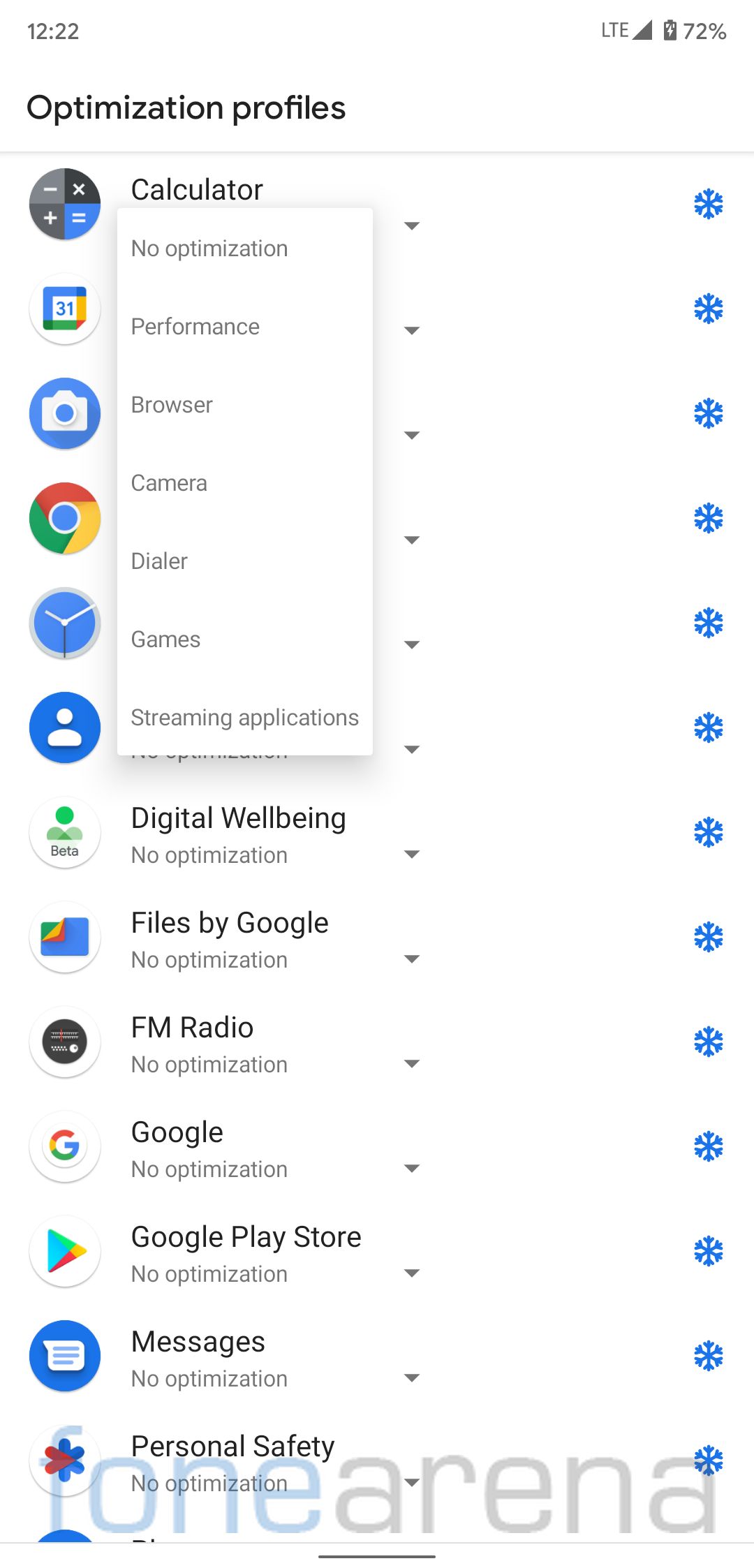A screenshot of a Google settings page on an Android phone displays various apps and services that are currently running, offering options for optimization. The screen shows icons for Calculator, Calendar, Photos, Google Chrome, Clock (including possible alarms), Digital Well-being, Files by Google, FM Radio, Google, Google Play Store, Messages, and Personal Safety. The page allows users to optimize these apps with choices like no optimization, performance optimization, browser optimization, camera optimization, dialer optimization, games optimization, and streaming applications optimization. Additional elements on the phone screen include LTE signal bars, battery level, and the current time, which is 12:22 PM. The interface suggests more settings and apps can be accessed by scrolling down, providing comprehensive control over the device's performance.